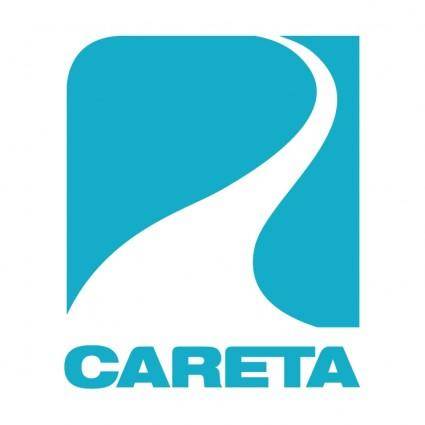The logo features a distinctive and minimalistic design with a combination of white and blue colors. It exists within a square frame that has rounded edges on the upper left and square edges on the other three sides. The primary element is a white, winding path that begins thick at the bottom of the square and gradually narrows as it meanders upward, first curving slightly to the right and then to the left. This path is set against a sky-blue background that occupies the left and right sides of the square. Directly below the path, at the very bottom of the square, is the text "CARETA," spelled out in bold, thick, uppercase blue letters. Notably, the "E" and "T" in "CARETA" are uniquely merged at the crossbar, creating an eye-catching stylistic touch. The overall background of the logo itself is a clean white, making the blue and white elements stand out prominently. This logo exudes simplicity and elegance, with the winding path and bold text suggesting a theme of guidance or direction, likely representing the brand identity of Careta.